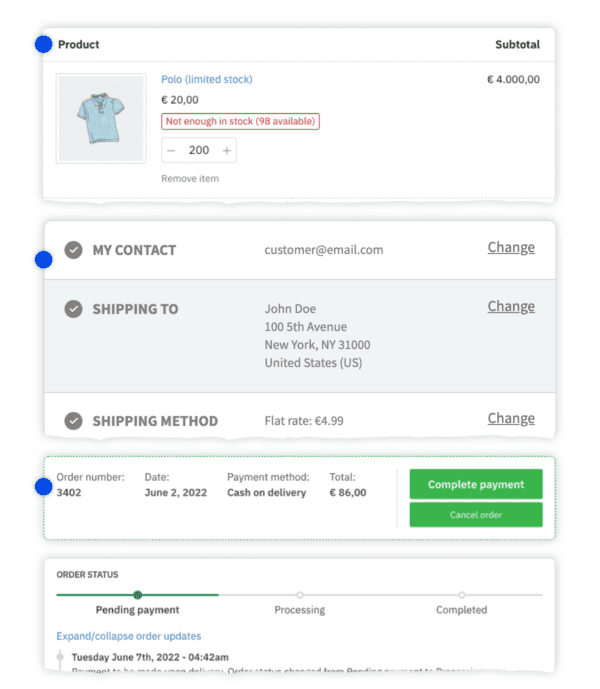Screenshot: Online Purchase Attempt for 200 Polo Shirts

Detailed description:

The screenshot captures an online purchase attempt from a retail website. The focus is on a polo shirt, which is currently listed as being in limited stock, with an available quantity of only 98 units. The shirt is priced at approximately 20 euros each. The individual attempts to purchase 200 polo shirts, resulting in a subtotal of around 4000 euros; however, the transaction is restricted due to insufficient stock.

Key details in the screenshot include an automated email address in place of the individual's contact details and a placeholder shipping address: John Doe, 105th Avenue, New York. This suggests the real shipping information has yet to be entered. The shipping method chosen is a flat rate of 4 euros and 99 cents. 

Further, the order number is identified as 3402, with a transaction date of June 2nd, 2022. The payment method specified is cash on delivery, amounting to a total of 86 euros. At the time of the screenshot, the order status is marked as 'pending for payment,' indicating the transaction is still in the processing stage and nearing completion.